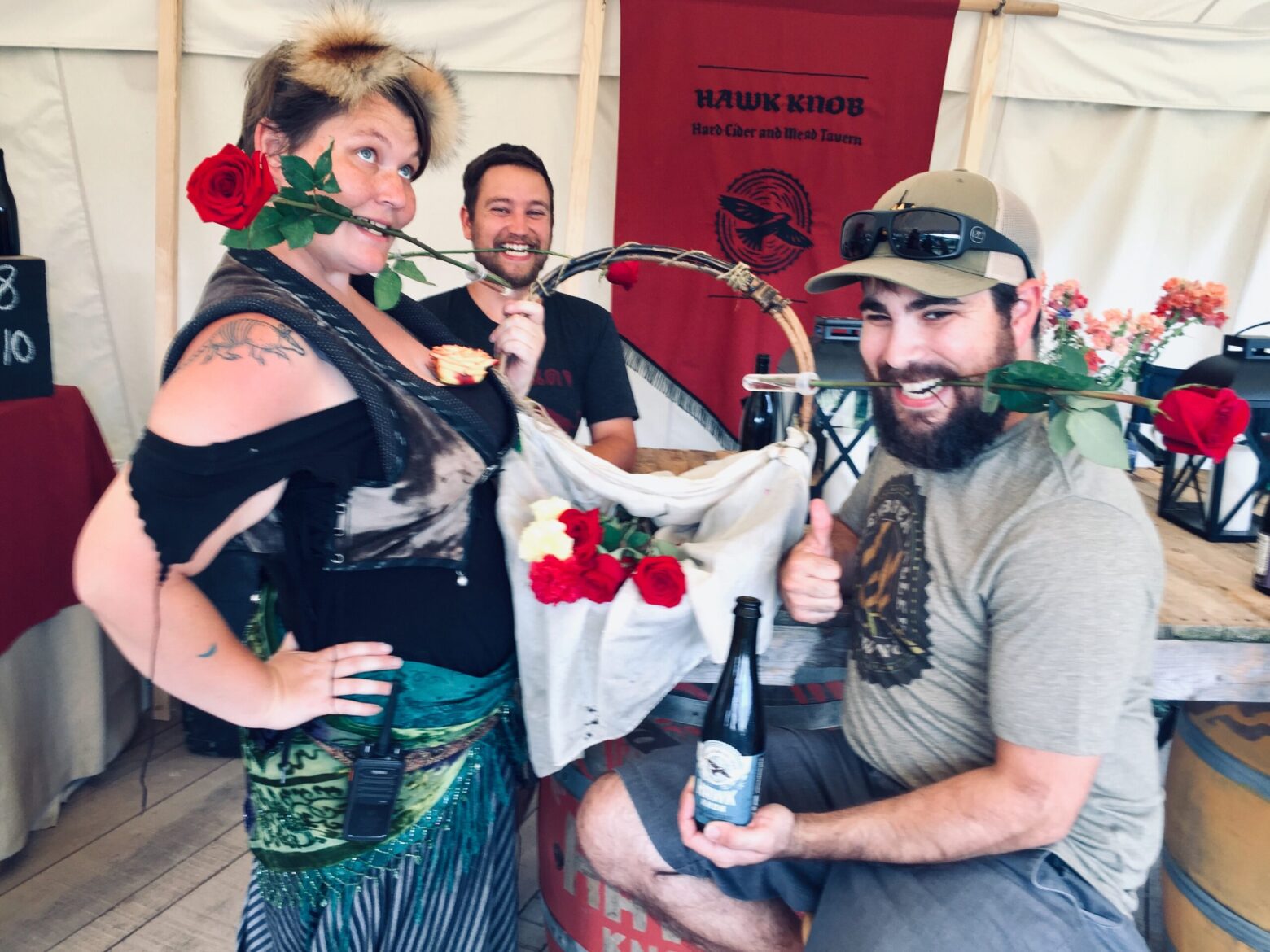In the photograph, three people are the focal point against a backdrop of what appears to be a white tent or canopy with wooden supports and a striking red banner. The banner, prominently hanging in the middle, reads "Hawk Knob" in bold black letters, with "Hard Cider and Mead Tavern" written underneath. There is a circular logo featuring a hawk in front of a wooden log or saw blade design, which also seems to be on the bottle one man is holding.

On the left stands a woman with short dark brown hair streaked with blonde, wearing a black off-the-shoulder cut-off t-shirt, a vest, and a vibrantly colored green, turquoise, and teal sarong-style skirt. She has a rose held between her teeth, one hand on her hip, and is possibly holding a walkie-talkie. Adorning her head is a pom-pom style headband. 

Behind her is a man smiling with light facial hair, also holding a rose in his teeth. He is casually dressed in a black t-shirt. The pair is connected by a basket filled with roses that she holds between them.

To the right, another man sits, leaning against a table that holds the rose basket. He is slightly chubby, with a thicker dark beard and hair, wearing a tan baseball cap with sunglasses perched on the brim, a gray t-shirt, and gray shorts. He, too, has a rose between his teeth and is holding a bottle of an alcoholic beverage while giving a thumbs-up gesture and smiling. 

The group exudes a playful, buoyant atmosphere set against the detailed backdrop, enhancing the photograph’s lively and festive feel.